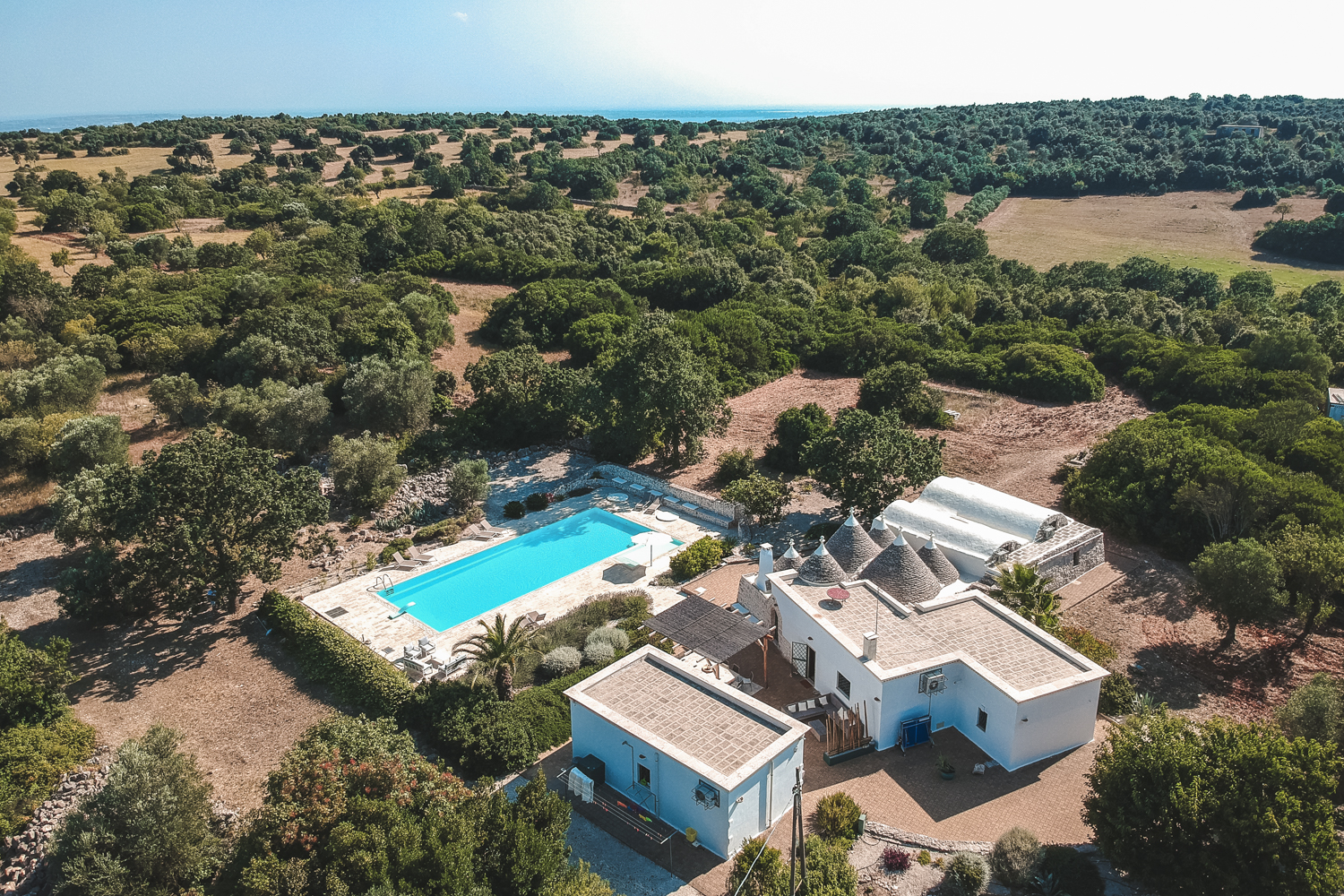This aerial photograph captures a secluded property set in a dry, desert-like environment, possibly in areas akin to Las Vegas or parts of California. The landscape is sparse with short, scrubbier trees and rocky terrain stretching into the distance, underscoring the isolation of the property. At the center of the image sits a main house, marked by unusual spiral cone decorations on its flat-tiled roof. There are two additional structures adjacent to the main house: one resembling a vertical Tetris piece and the other a basic rectangle, possibly serving as a guest or pool house. Each structure is single-story and painted white with brick roofing. Behind the buildings is a large, inviting in-ground swimming pool surrounded by marble stonework and a bit of fencing, detailed with an umbrella, a few chairs, and tables. Nearby, several palm trees add a touch of green to the otherwise arid scene. The overall impression is one of a thoughtfully designed, isolated desert retreat—complete with amenities for relaxation under the expansive sky.